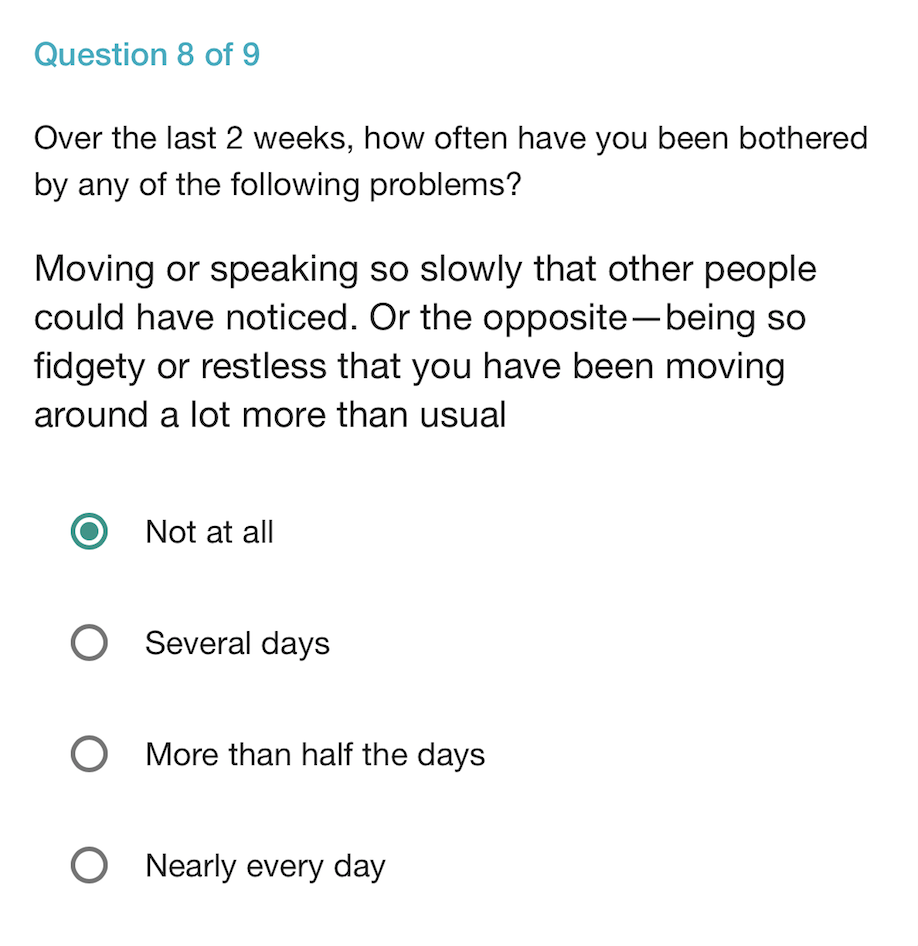This image is a detailed screenshot of a question from a personality test or mental health assessment, likely designed to evaluate symptoms of depression. The screenshot features a clean white background without any borders. At the top left, blue text highlights the progress of the assessment, indicating "Question 8 of 9." Below this, in prominent black font, the question asks, "Over the last two weeks, how often have you been bothered by any of the following problems? Moving or speaking so slowly that other people could have noticed. Or the opposite, being so fidgety or restless that you have been moving around a lot more than usual."

Four response options are provided beneath the question, each preceded by a grey circle:
1. Not at all
2. Several days
3. More than half the days
4. Nearly every day

The first response option, "Not at all," is selected, distinguished by a blue-outlined circle with a white inside circle and a blue center.

This question appears to be part of an assessment tool aimed at identifying symptoms indicative of depression, specifically evaluating psychomotor retardation or agitation.